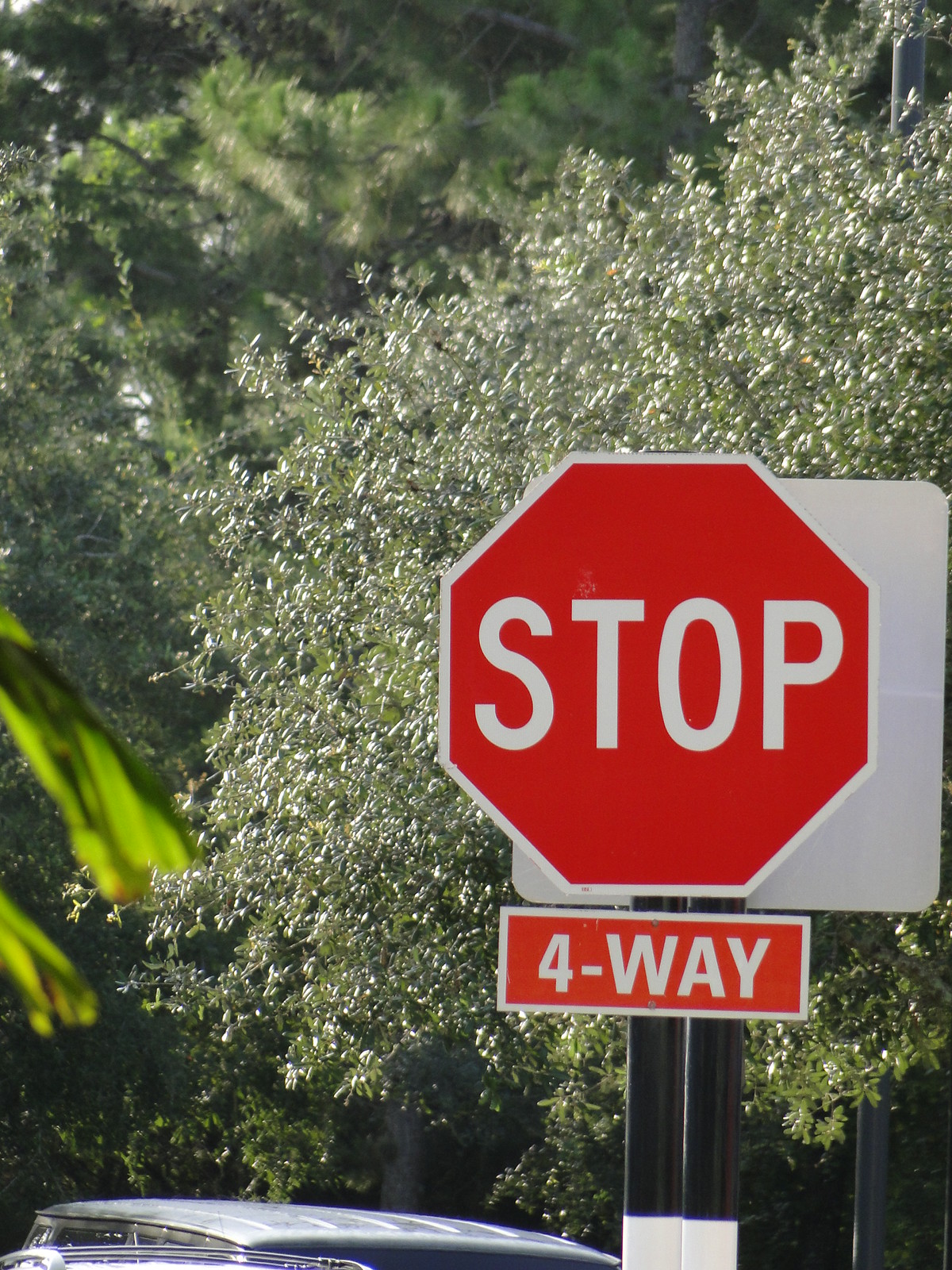This vibrant color photograph primarily features a large, red, hexagonal stop sign prominently positioned towards the middle and lower part of the image. The stop sign is outlined in white, with the word "STOP" boldly displayed in white letters against the red background. Below the main sign is a smaller rectangular sign, also red with white outlines, reading "FOUR WAY." Both signs are mounted on a black metal pole. 

In the background, various trees fill the scene, their green foliage creating a lush backdrop. On the right side of the image, there's a big tree with green and white leaves, while more trees with both light and dark green leaves can be seen towards the left and upper parts of the image. These leaves are sunlit but the stop sign remains unlit. Partially visible at the bottom of the photograph is the top or roof of a gray car. Additionally, the white back of a square sign facing the opposite direction is visible, attached to the same post as the stop sign. 

Overall, the backdrop of trees and the slightly obtrusive car frame the central subject of the stop sign, making it the focal point of this outdoor scene.